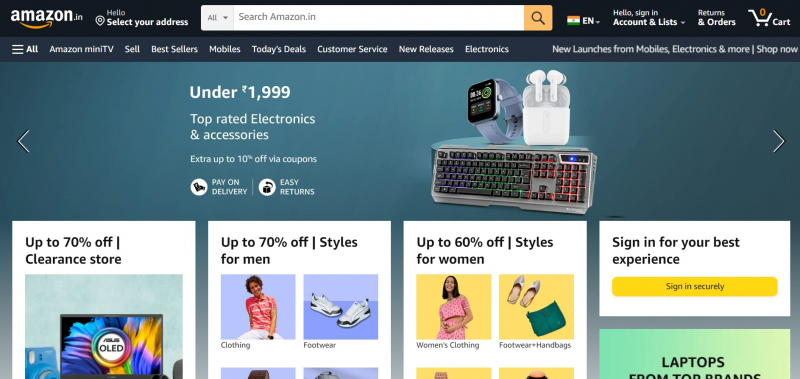This is a detailed description of an Amazon webpage image. The image is a wide rectangle, approximately twice as wide as it is tall. The upper fifth of the image features a black band with white text. In the upper left corner, the Amazon logo with its characteristic curved orange arrow is displayed. To the right of the logo are the words "Hello, select your address" in white.

Next is the Amazon search bar, immediately followed by an orange search icon. To the right of the search icon is a small flag in orange, white, and green colors, next to a white drop-down box with the letters "EN" in capital letters. Further to the right, white letters spell out "Hello, sign in, account, and lists.” This is followed by "Returns & Orders" and a shopping cart icon with an orange zero, accompanied by the word "Cart" to its right.

Beneath this black band, there's a series of menu selections stretching across the entire width of the image. Following this is a wide teal blue band with white text that reads: "Under $1,999, top rated electronics and accessories. Extra up to 10% off via coupons." Below that, there are two options, "Pay on Delivery" and "Easy Returns," each accompanied by a white circular logo with a black icon to the left. 

To the right within the teal blue box, an image of various electronic equipment including what appear to be earbuds, an Apple Watch, and a keyboard is displayed.

Below the teal blue section, there are four white boxes containing pictures and text. The leftmost box advertises "Up to 70% off Clearance Store," featuring an image with a blend of pale blue, purple, orange, and red colors, possibly resembling a TV screen. The second box to the right promotes "Up to 70% off Styles for Men" with a lavender background, showing a young man in a red and white shirt and white pants, and another image of tennis shoes. The box is labeled with "Clothing" and "Footwear."

The third box similarly promotes "Up to 60% off Styles for Women," displaying images of a young woman in a pinkish-red dress against a yellow background, and another image showing shoes and a green handbag, labeled "Women's Clothing" and "Footwear & Handbags." 

The rightmost box encourages users to "Sign in for your best experience" with a long yellow rectangle below it saying "Sign in securely." There is a light green square underneath with "Laptops" written in black letters, though only the top part of the square is visible, the words "From Top Brands" partially showing beneath.